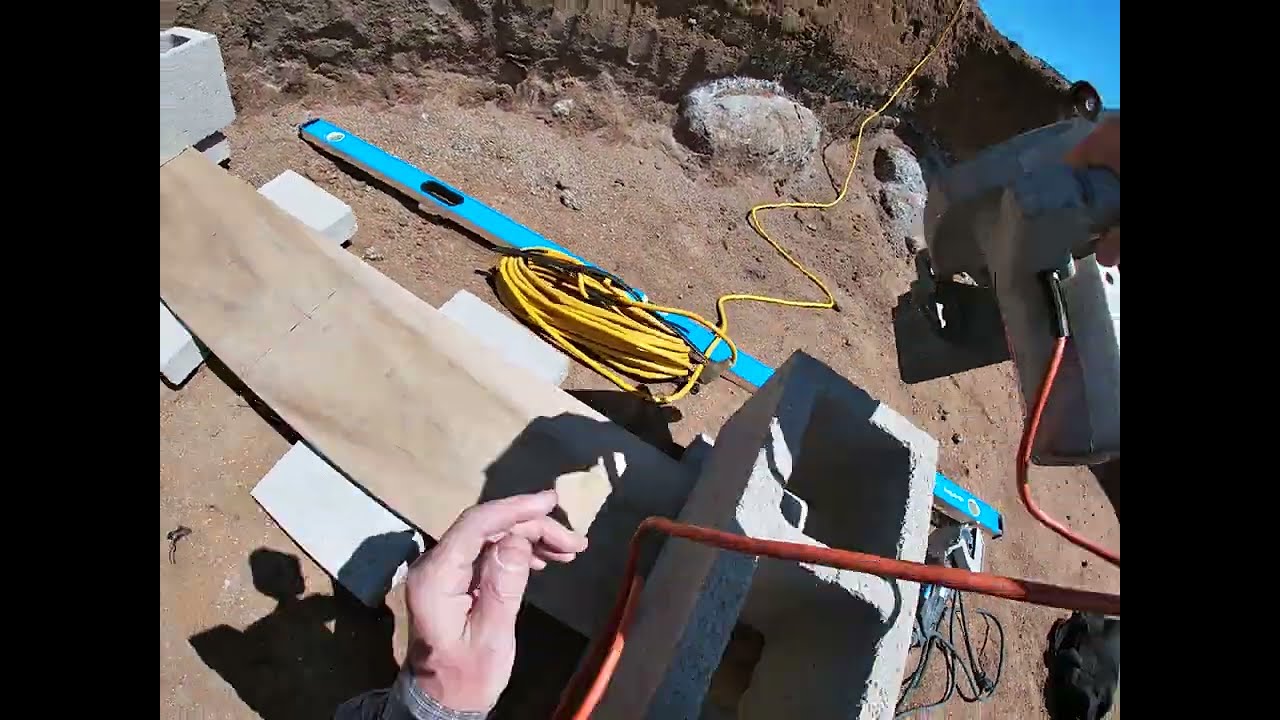The horizontally aligned rectangular photo showcases a person's hands engaged in construction or repair work on a rocky and dirt-strewn ground. The image is framed by narrow vertical black borders on both sides. The scene features a clear blue sky in the upper right corner, with the top edge dominated by a textured, brown rock cliff. The central and lower sections of the photo display mostly flat land covered in dirt and small rocks. 

In the lower part of the image, towards the left, a left hand clad in a plaid long-sleeve shirt is visible, apparently about to grab a metal bar or cord that runs across the frame to connect to a handheld tool resembling a sander. An orange cord connects to this tool, and a glimpse of fingertips can be seen holding it in the upper right corner, though it is unclear if the hand belongs to the same person.

Scattered around the workspace are several building materials, including a coiled yellow extension cord, which snakes up the side of the cliff, and a cinder block or concrete slab. A blue spirit level lies on the ground near the tool, further suggesting the activity involves precise construction or measurement. The scene offers a first-person perspective, as if viewed from a camera attached to a helmet, detailing an outdoor worksite where the individual appears to be building or repairing a structure in the dirt.